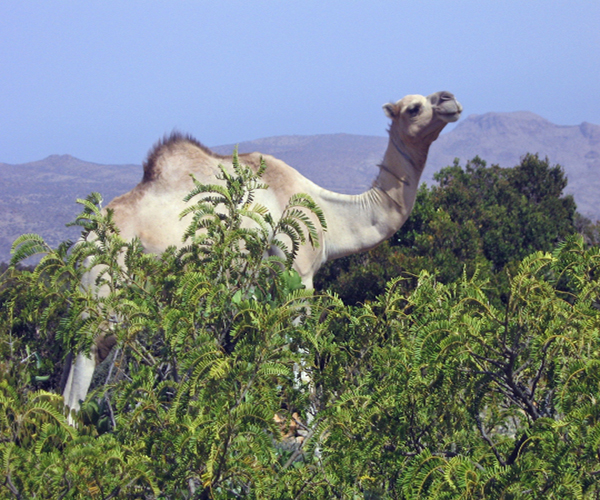In this captivating desert scene, the viewer is treated to an intriguing visual illusion. The background is dominated by majestic mountains under a blue sky tinged with gray, suggestive of either cloudy weather or pollution. In the foreground, verdant greenery — comprising what initially seem to be full-sized tropical trees — adds a splash of life to the arid landscape. However, the true centerpiece of the image is a two-humped, pale camel. Due to a clever use of perspective, the camel appears to tower over the "trees," giving the impression of a gargantuan beast capable of devouring an entire forest, with humans being mere crumbs of a snack in comparison.

Upon closer inspection, one realizes that the "trees" are, in fact, bushes and large weeds, creating an optical illusion that makes the camel seem impossibly large. This whimsical forced perspective playfully tricks the eye, suggesting the camel is striding above a canopy when it is actually standing among much smaller vegetation. The juxtaposition of scale between the camel and its surroundings creates a striking and memorable image, blending natural beauty with a touch of surreal, giant-sized fantasy.